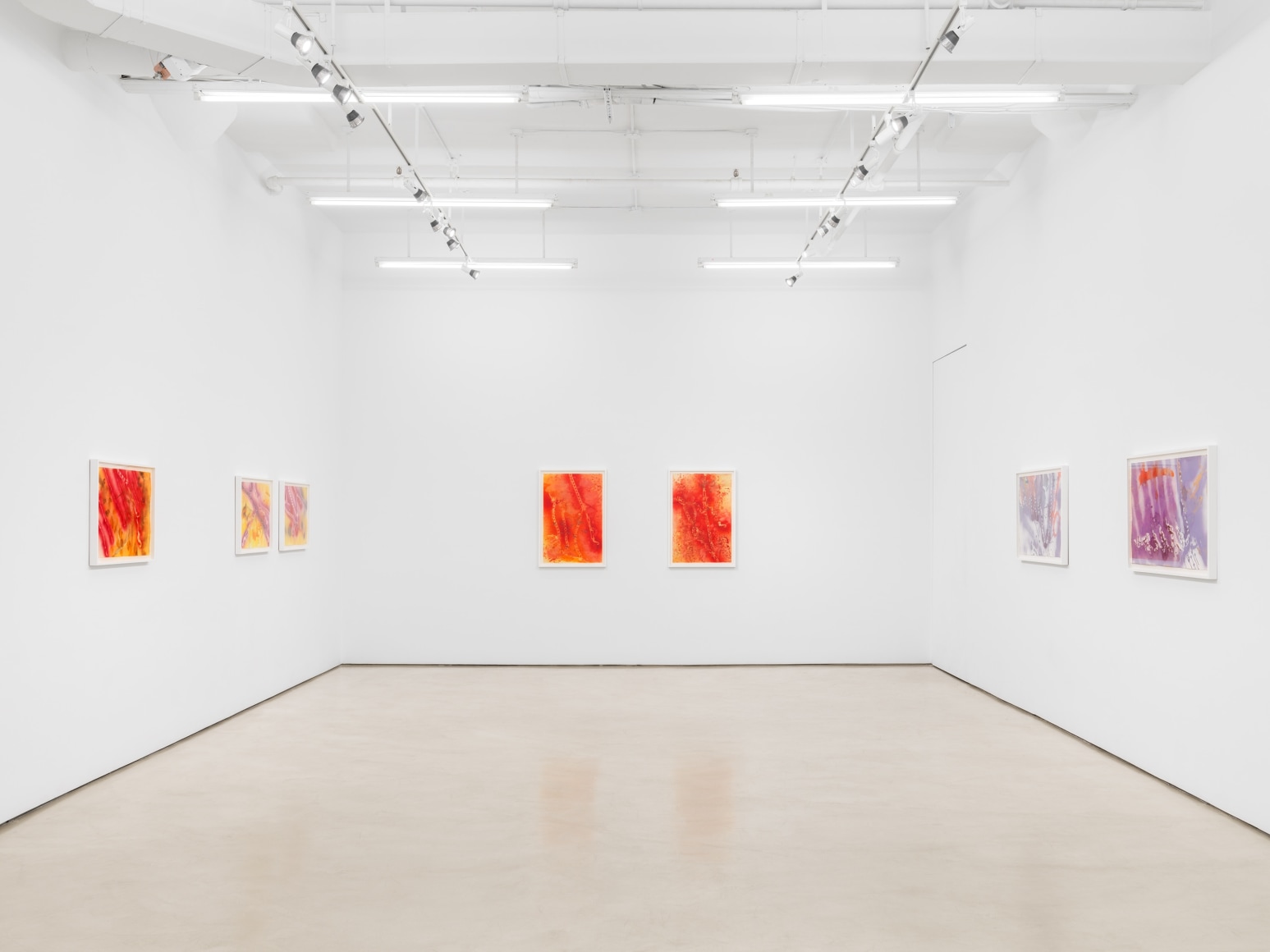The image depicts an extremely stark and bare art gallery featuring white walls, a lilac floor, and a white ceiling illuminated by six ceiling-mounted LED lights and additional spotlights on both the left and right. There are seven pieces of artwork in total, all framed in white and characterized by abstract splatter designs with vibrant colors. 

On the back wall, there are two similar pieces showcasing an orange, reddish, and yellow splatter pattern, resembling a pair. The left wall displays three frames: the one furthest left mirrors the orange and red splatter design of the back wall pieces, while the two closer together exhibit yellow and purple splatter patterns. On the right wall, two frames feature abstract designs dominated by purples and blues, with one containing a touch of orange. The overall sterility and simplicity of the space, combined with the consistent use of vibrant, abstract art, highlight a minimalistic and modern aesthetic typically found in contemporary art galleries.